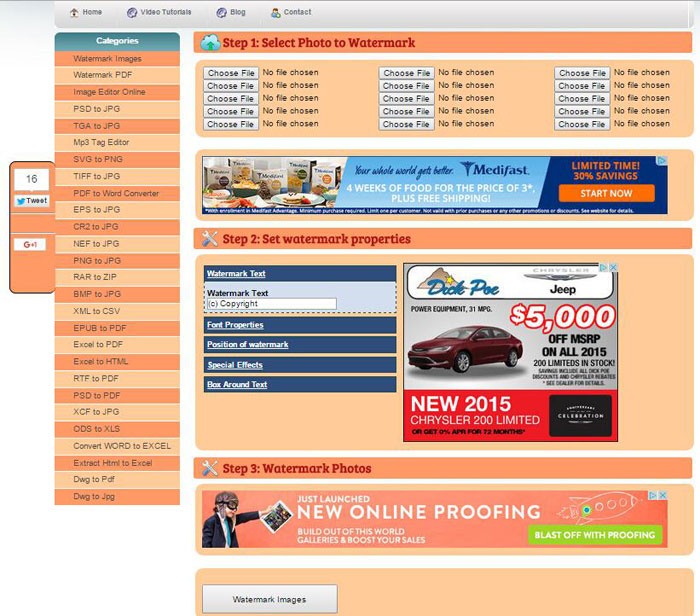In this image, we see a detailed screenshot of a website, likely a tool for watermarking images and managing files. At the very top, there is a gray navigation bar with the menu options: Home, Video Tutorials, Blog, and Contact.

On the left-hand side, a sidebar features a section header labeled "Categories." Below this are several rectangular buttons alternating between bright and pastel orange, each labeled with different options for file conversions and editing. The options listed are: Watermark Images, Watermark PDF, Image Editor Online, PSD to JPG, TGA to JPG, MP3 Tag Editor, SVG to PNG, TIFF to JPG, PDF to Word Converter, EPS to JPG, CR2 to JPG, NEF to JPG, PNG to JPG, RAR to ZIP, BMP to JPG, XML to CSV, EPUB to PDF, Excel to PDF, Excel to HTML, RTF to PDF, PSD to PDF, XCF to JPG, ODS to XLS, Convert Word to Excel, Extract HTML to Excel, DWG to PDF, and DWG to JPG. Adjacent to these options is a small orange box displaying the number 16, with icons for Twitter (Tweet) and Google Plus (G+1).

To the right of the sidebar, the main section of the page begins with an orange header labeled "Step 1: Select Photo to Watermark." Below this header are five columns of three gray buttons each, totaling fifteen buttons labeled "Choose File," accompanied by the text "No File Chosen."

Further down is another orange box containing a blue advertisement. The ad promotes a food delivery service, stating: "Your whole world gets better, mighty fast. Four weeks of food for the price of three, plus free shipping. Limited time, 30% savings. Start now."

Below this ad, another orange header marks "Step 2: Set Watermark Properties." This section includes several blue boxes with the labels: Watermark Text, Watermark Text, See Copyright, Watermark Properties, Position of Watermark, Special Effects, and Box Around Text. To the right of these elements is an ad for "Dick Poe Jeep," featuring a picture of a car and a promotion: "$5,000 off MSRP off all 2015 200 Limiteds in stock." Below the ad, a red box highlights, "New 2015 Chrysler 200 Limited."

Towards the bottom, another orange header indicates "Step 3: Watermark Photos." This section is followed by an ad featuring a child wearing airplane goggles and a hat, holding up a picture. The ad encourages viewers to use their new online proofing service: "Just Launched, New Online Proofing, Build Out of This World Galleries and Boost Sales. Blast off with proofing."

The image concludes with an orange bar containing a gray box labeled "Watermark Images."